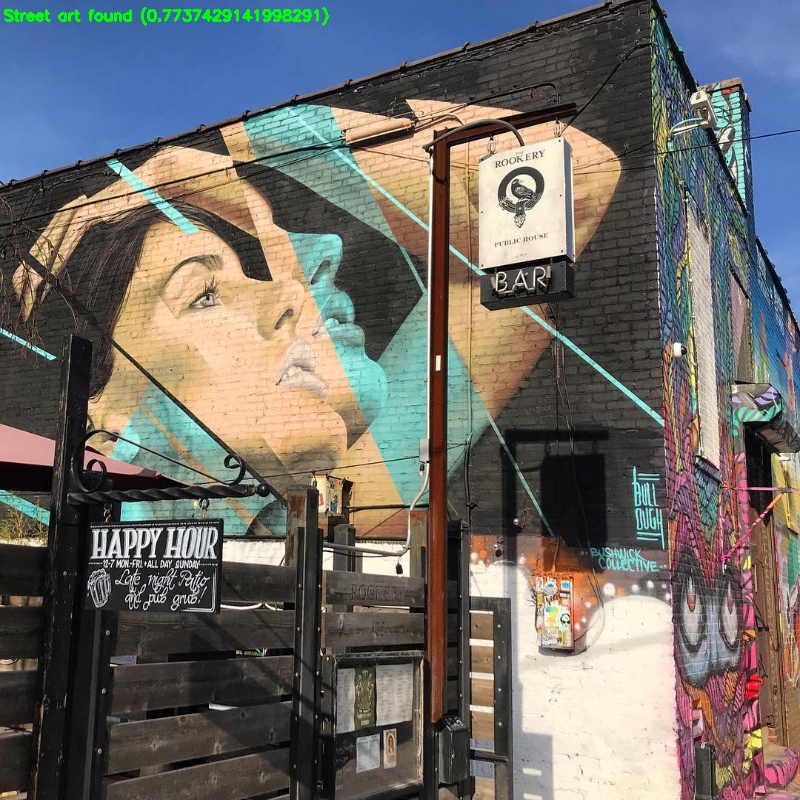The exterior of the Rookery Public House bar features a vibrant, expansive mural that wraps around the side and front of the building. The focal point of the mural is a striking portrait of a woman with dark hair, raising her left arm over her head. Her face is partially reflected in diagonal blue streaks that add a dynamic touch to the artwork. Alongside her, another woman's nose, lips, and chin emerge, also painted with a bluish hue over a tan base. The mural showcases a plethora of colors, including turquoise, blue, purple, pink, orange, and red, creating a lively and eclectic atmosphere.

On the left side of the building, a wooden fence encloses a yard, adorned with a black sign bearing white text. It announces happy hour from 12 to 7 PM, Monday through Friday, and all day on Sunday. Below this, another sign reads "late night patio and pub grub!" 

Additionally, the bar's name, "Rookery," is displayed prominently in neon tubes on a steel beam. To the side and partially towards the back of the building, "Bushwick Collective" and "Bulldell" are inscribed in blue paint, integrating seamlessly into the mural's vibrant color scheme. The overall scene captures a lively street art motif, with a blend of detailed portraits and abstract graffiti.